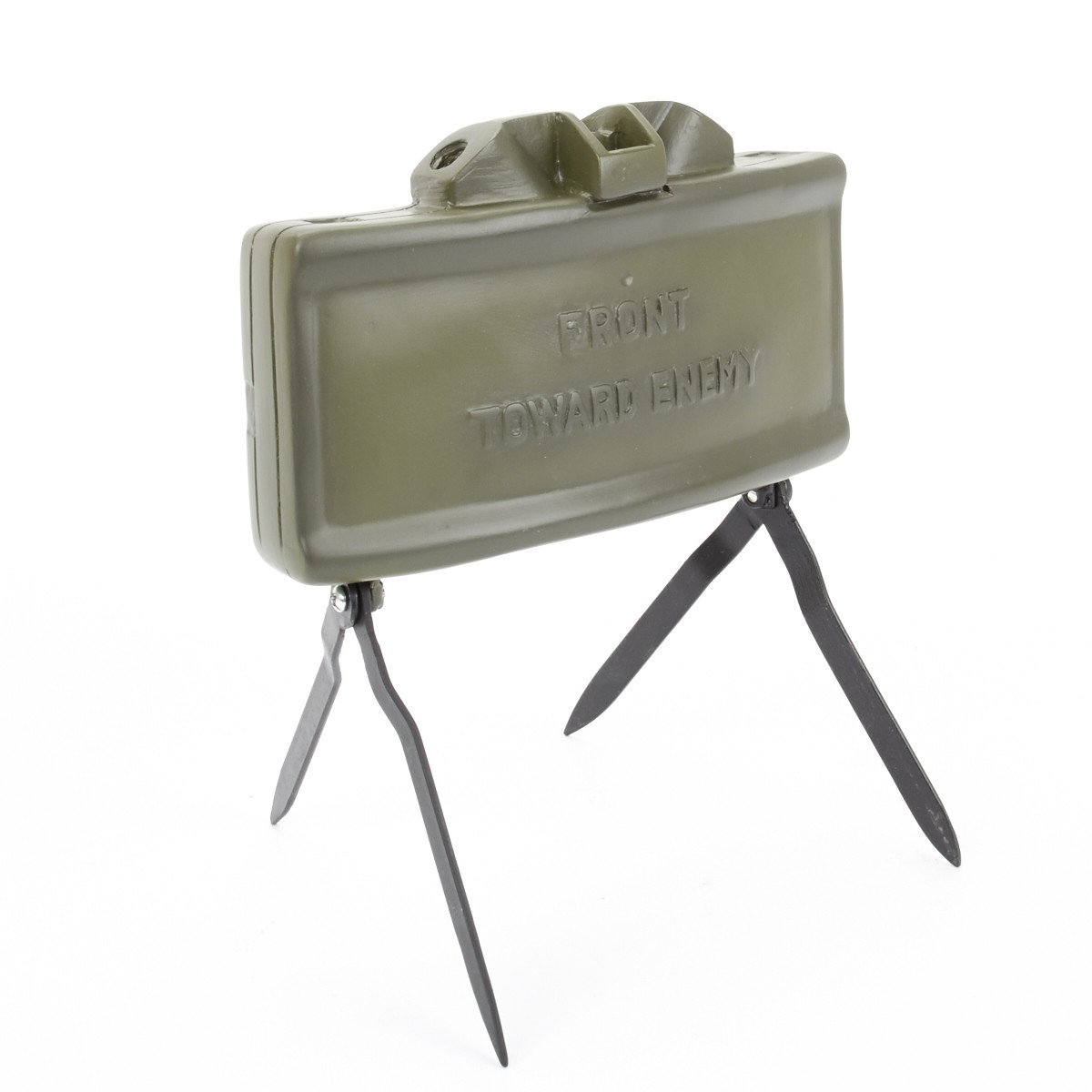This image depicts what seems to be a military-related device, likely a mine or explosive, known for its distinctive design and warnings. The object is a rectangular box made of hard plastic in a greenish-gray, or olive-green, color, set at an angle of approximately 35 degrees. The front of the box prominently features the raised text "Front Toward Enemy," ensuring clear orientation for use. The device is supported by two dark gray, upside-down V-shaped metal legs, which resemble sharp, scissor-like stands, presumably designed to anchor the device firmly into the ground. At the top of the box are three molded bumps, with the leftmost bump featuring a circular hole. Despite its menacing functionality, the overall appearance is plain and utilitarian, emphasizing its purpose rather than aesthetics. The contextual lack of background details leaves the actual size of the device ambiguous, contributing to its enigmatic presence in the image.